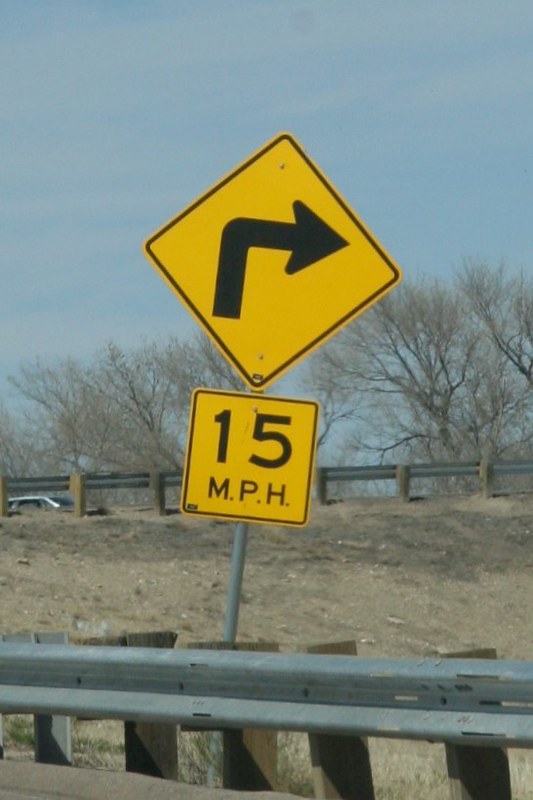In this photograph, a prominent yellow and black sign indicates a sharp right turn with a suggested speed limit of 15 miles per hour. The immediate foreground features sturdy guard rails for safety, with additional guard rails visible on a distant road. The background is adorned with trees that have shed their foliage, suggesting an autumn or winter setting. The sky overhead is a clear yet muted shade of blue, adding to the seasonal atmosphere. On the left side of the image, the top of a car is visible, either parked or making the right turn indicated by the sign. The overall composition highlights the winding road and the precautions in place for drivers navigating this sharp turn.